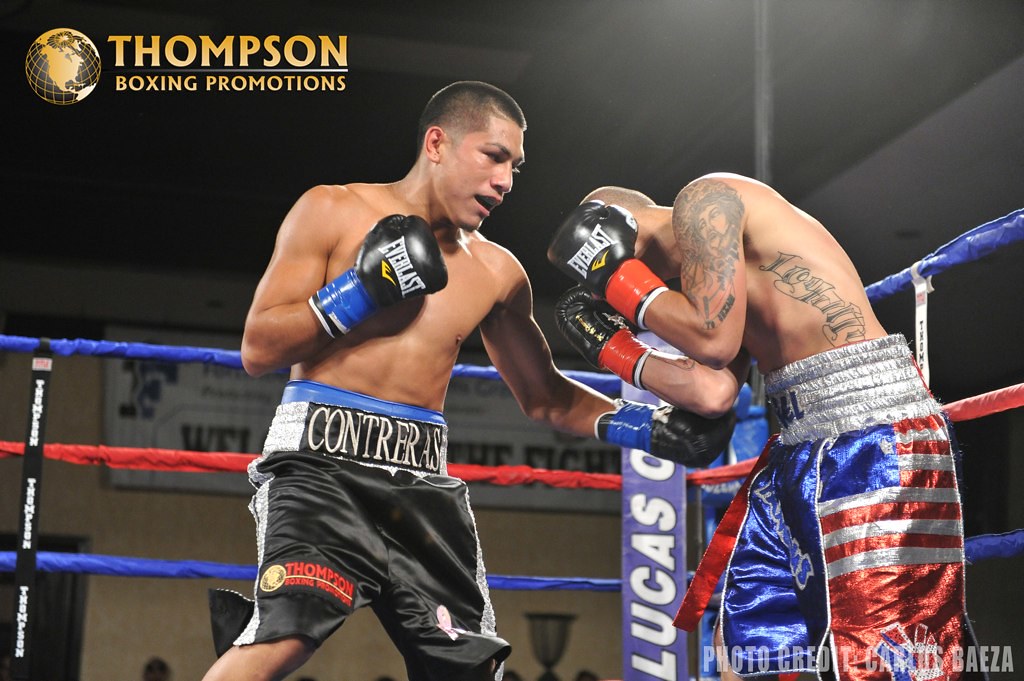In this detailed photograph of an intense boxing match, two opponents are captured mid-action in the center of a ring. The setting appears to be indoors, likely a gymnasium, as indicated by the surrounding elements. The boxer on the left is wearing black shorts with the name "Contreras" printed on the belt and black Everlast gloves. This fighter is executing a lead left punch aimed at the body while keeping his right hand cocked, but his chin remains exposed. The opponent on the right, distinguished by his American flag-themed shorts and heavily tattooed left arm and side, is crouched defensively with his hands protecting his head and elbows guarding his midsection.

The ring itself is vividly colored with red, white, and blue ropes arranged from top to bottom, and one of the ring corners bears the vertical inscription “Lucas Oil,” one of the sponsors. Above the action, in the top left corner of the image, a yellow text against a black background reads "Thompson Boxing Promotions" next to a black and gold globe featuring North America. At the bottom right, photo credit is given to Karats Beza. The visual palette of the image includes a range of colors such as red, white, blue, gray, tan, black, brown, orange, and yellow, contributing to the vibrant atmosphere of this high-stakes boxing bout.